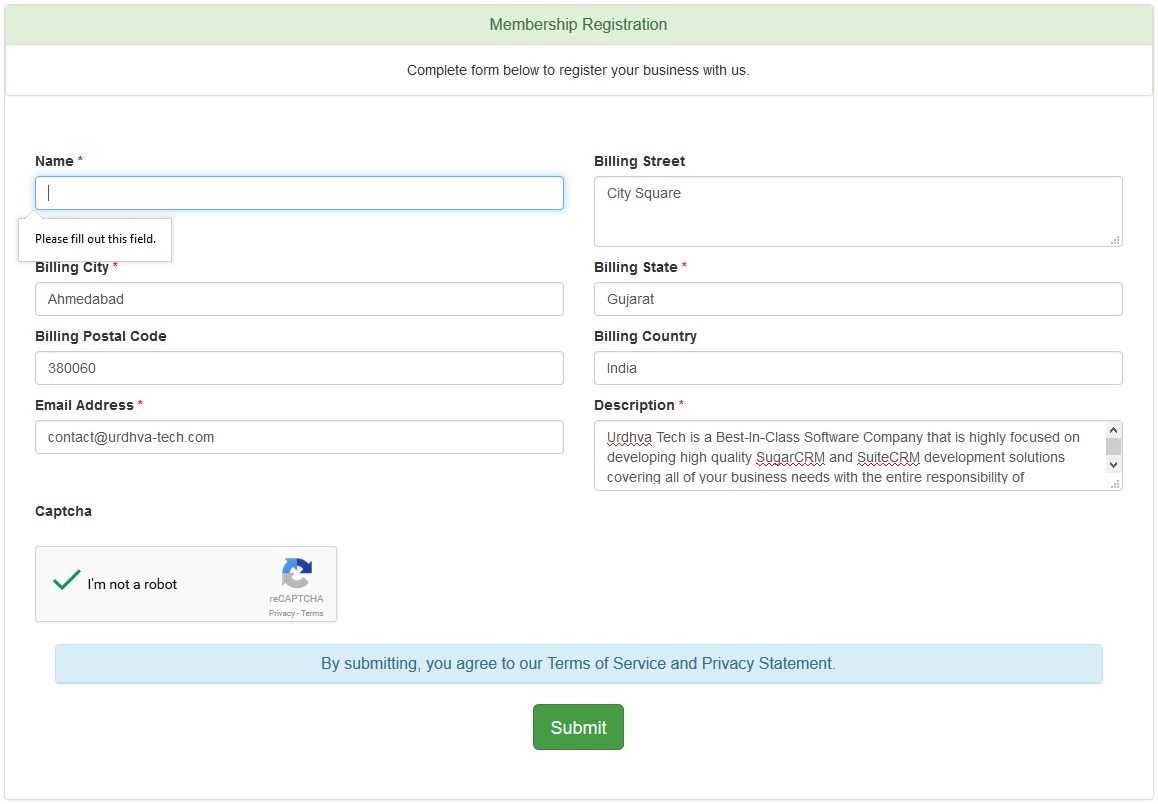Here is a detailed and cleaned-up caption for the image described:

---

This screenshot captures a website's membership registration page. At the top, a horizontal greenish rectangle features the heading "Membership Registration" in a striking dark green font. Directly below, another horizontal rectangle contains the instruction "Complete Form Below to register your business with us."

On the left side of the form, there is a field labeled "Name" with a red asterisk indicating it is required. The text "Please fill out this field" appears, emphasizing its mandatory nature. Beneath it, the bold, dark font label "Billing City" is followed by the text "AHMED." Additionally, the "Billing Postal Code" is listed as "3860," and an email address "contact@urdhva-tech.com" is provided.

The right side of the form details further billing information with headers in dark font, including "Billing Street," "Billing State," and "Billing Country." The respective entries are "City Square" for the street, "Gujarat" for the state, and "India" for the country. A description box is filled with relevant information.

At the lower left, a checked captcha box confirms "I'm not a robot." Just above a green submit button with white text, a statement reads, "By submitting, you agree to our terms of service and privacy statement."

---

This revised caption provides a detailed and organized description of the elements present in the image.